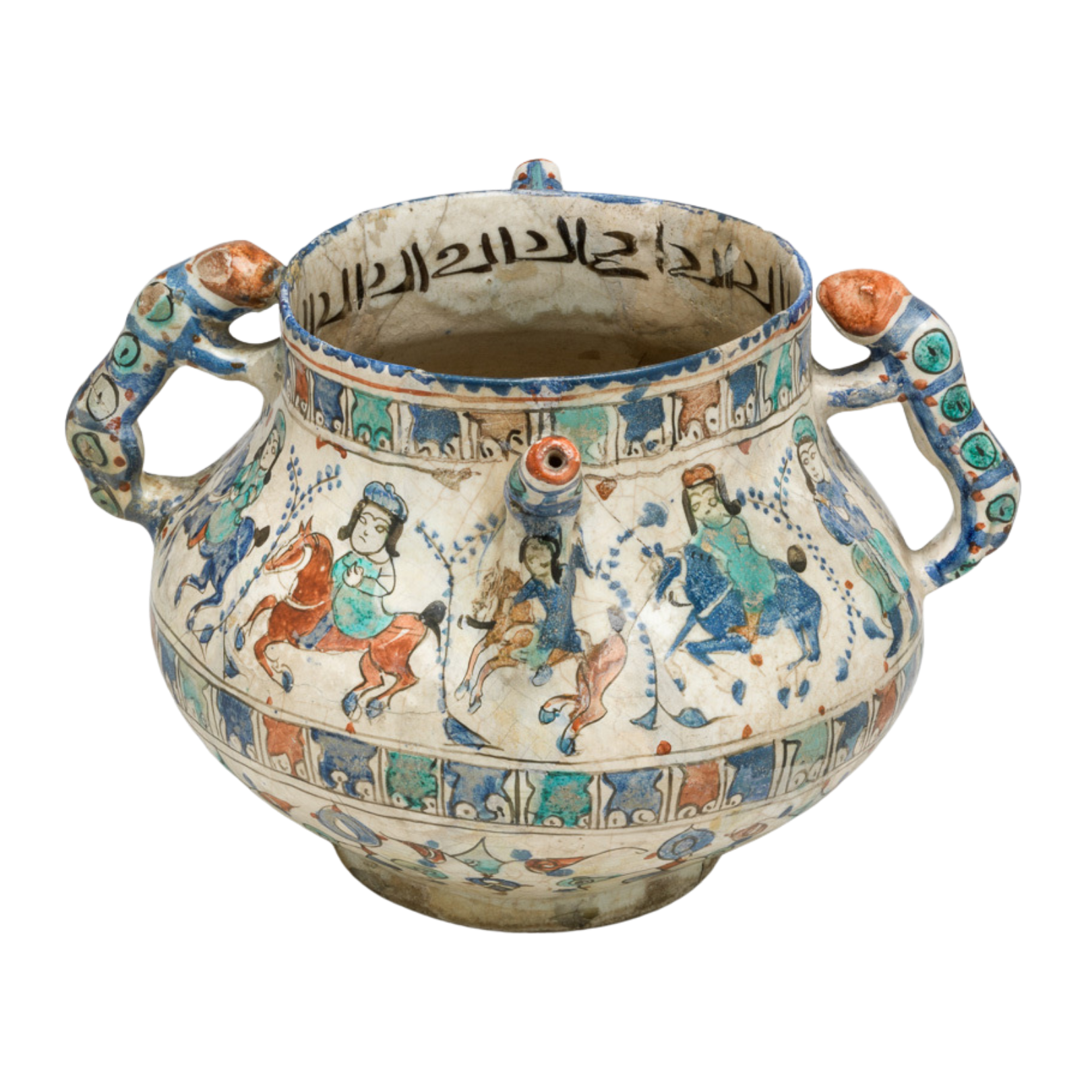The image features a single, distinctive, culturally significant piece of pottery, likely from India or Persia, given its ethnic aesthetics and intricate detailing. The pot, ancient and ceramic, exhibits a base color of cream beige with an array of colors including green, orange, brown, and blue. The surface is richly decorated with scenes of men riding horses, clad in traditional robes and hats, surrounded by various onlookers. The artwork extends across the entire circular body of the pot, integrating floral patterns and geometric designs featuring little square elements with eye-like features. The pot, reminiscent of both Asian and Middle Eastern craftsmanship, shows notable signs of age with visible cracks. On the internal rim, there are inscriptions in what appears to be Asian or Middle Eastern script. Handles on either side of the pot incorporate an ergonomically designed, animal-like form, accented with green circles and ornate red tips that almost reach the upper rim. The entire piece suggests great antiquity, likely several hundred years old, and stands against a simple white backdrop.